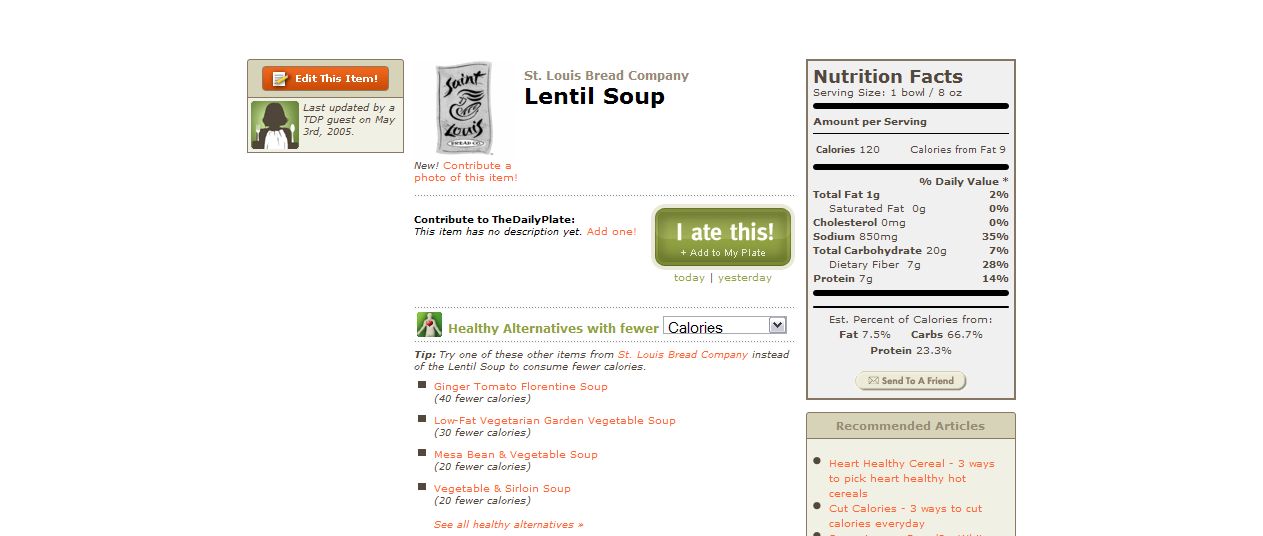This color image appears to be a screenshot from a diet-tracking website featuring a detailed breakdown of the nutritional facts for St. Louis Bread Company's Lentil Soup. On the left-hand side of the image, there is a small picture of what seems to be the front of the soup package, with the word "New" below it. The top left corner of the image is marked with "Edit this item" and notes that it was last updated by a TDP guest on May 3, 2005. 

Underneath, it introduces the Lentil Soup and includes an option to "Contribute a photo of this item" along with "Contribute to the daily plate." There is also a green button labeled "I ate this" allowing users to add the item to their dietary log. Beneath this, there's a section for "Healthy alternatives with fewer calories," suggesting other soups like Ginger Tomato Florentine Soup (40 fewer calories), Low Fat Vegetarian Garden Vegetable Soup (30 fewer calories), Mesa Bean and Vegetable Soup (20 fewer calories), and Vegetable and Sirloin Soup (20 fewer calories).

The Nutrition Facts section is on the right-hand side, displaying information for a serving size of one bowl (8 ounces): 120 calories, 9 of which are from fat. Additional nutritional details include 1 gram of total fat, 0 grams of saturated fat, 0 milligrams of cholesterol, 850 milligrams of sodium, 20 grams of total carbohydrate, 7 grams of dietary fiber, and 7 grams of protein. Estimated percentages of calories are provided as well: 7.5% from fat, 66.7% from carbs, and 23.3% from protein.

At the bottom, there are links to recommended articles such as "Heart Healthy Cereal: Three Ways to Pick Heart Healthy Hot Cereals" and "Cut Calories: Three Ways to Cut Calories Every Day." An icon featuring an envelope suggests users can "Send to a friend."